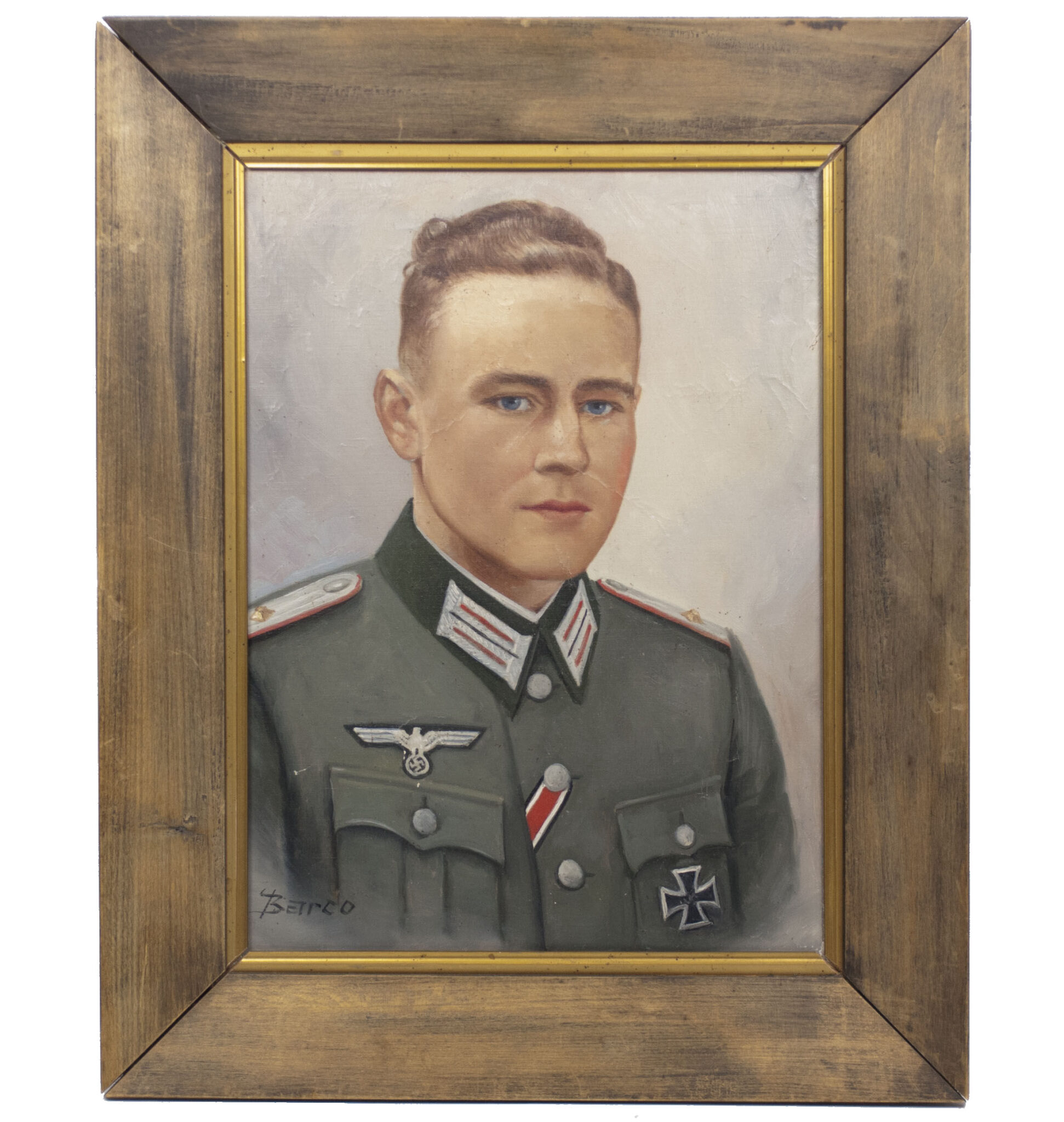The image captures a highly detailed, realistic painting of a young German soldier from World War II, dressed in a distinctive gray or forest green German military uniform. The soldier, who is fair-skinned with bright blue eyes and wavy blonde or reddish-brown hair, displays a stern expression. His uniform features significant insignia, including a German eagle on the right breast and a German cross on the left, as well as epaulettes that suggest a rank higher than private. Additional indicators of his rank include gold emblem markers on his shoulders and red stripes around his neck. The painting is signed by an artist named Barco, with the signature located at the bottom left corner. The artwork is housed within a simple wooden frame with visible grain patterns, which is painted brown. An inner lining of the frame appears to be brass or painted to resemble copper or gold, adding a subtle decorative touch. The piece is a photograph of a painting, capturing the essence and regalia of a Nazi officer.